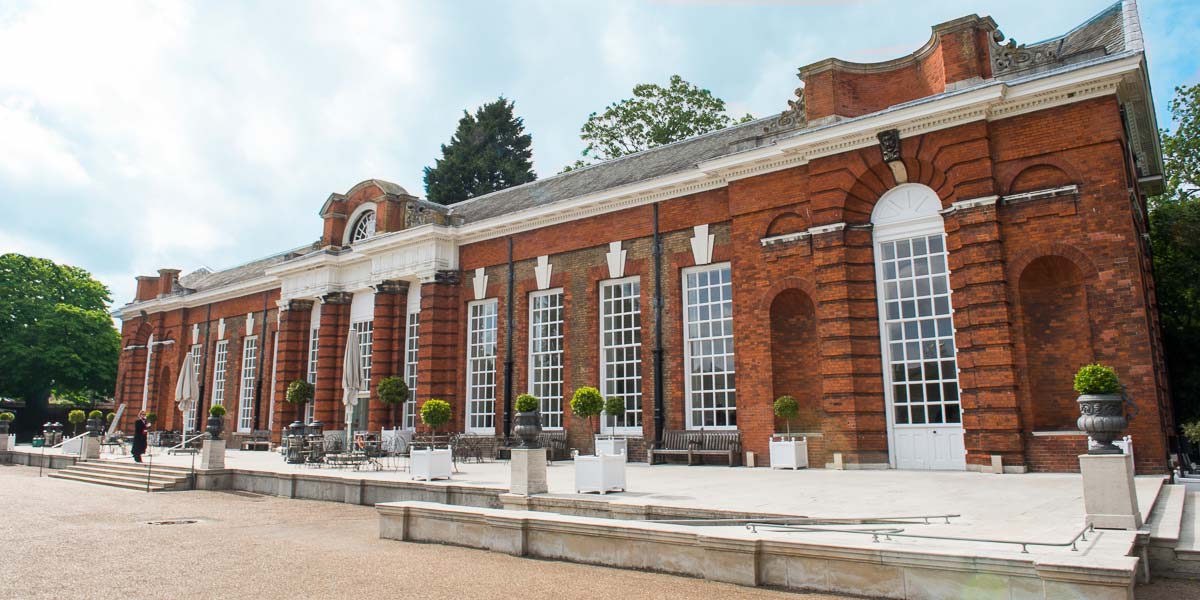The image depicts a stunning one-story red brick building, possibly serving as a catering hall or business center, set against a bright, partially cloudy sky. Its elegant architecture features large, floor-to-ceiling windows with white grid-patterned panes, including prominent archway windows at the front. The paved area, potentially made of cement, interlocking brick, or gravel, is lined with planters containing small trees with long stems and puffy, lollipop-like tops. Adding to the charm, there are red and white planters arranged periodically. The building is surrounded by very high trees on the side, back, and front, creating a lush backdrop. At the forefront, a woman dressed in black is descending cement stairs leading to a spacious cement platform adorned with various potted plants and furnished with outdoor umbrellas atop chairs, enhancing the inviting atmosphere.